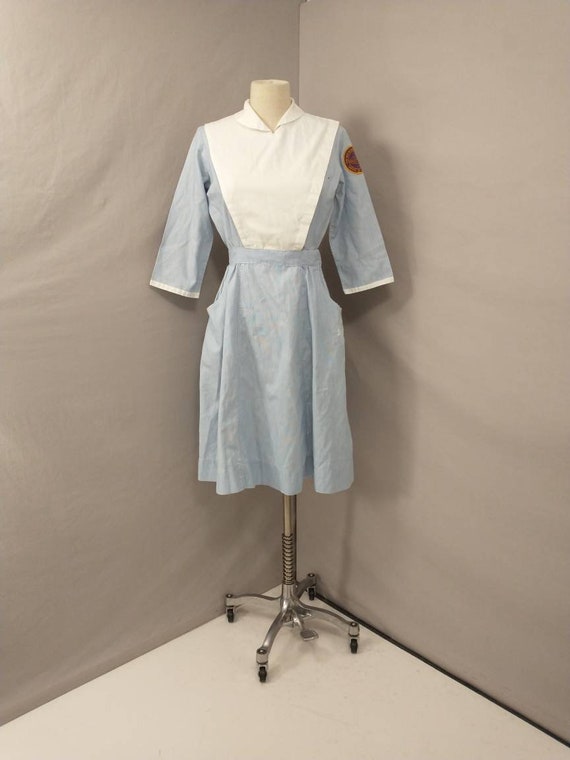The image depicts a close-up of an old-fashioned medical or nurse's uniform worn by a partial mannequin. The mannequin, which only reveals its neck protruding from the garment's collar, stands on a metallic rod-like platform with four black wheels. The uniform is a one-piece dress that is predominantly blue with white accents on the chest area and sleeves, ending roughly at the elbows. The garment features a small folded collar, two pockets, and a knee-length skirt. Notably, there is a burgundy or red patch with gold accents on one of the sleeves. This entire setup is positioned in the corner of a room with gray walls and a light gray floor.